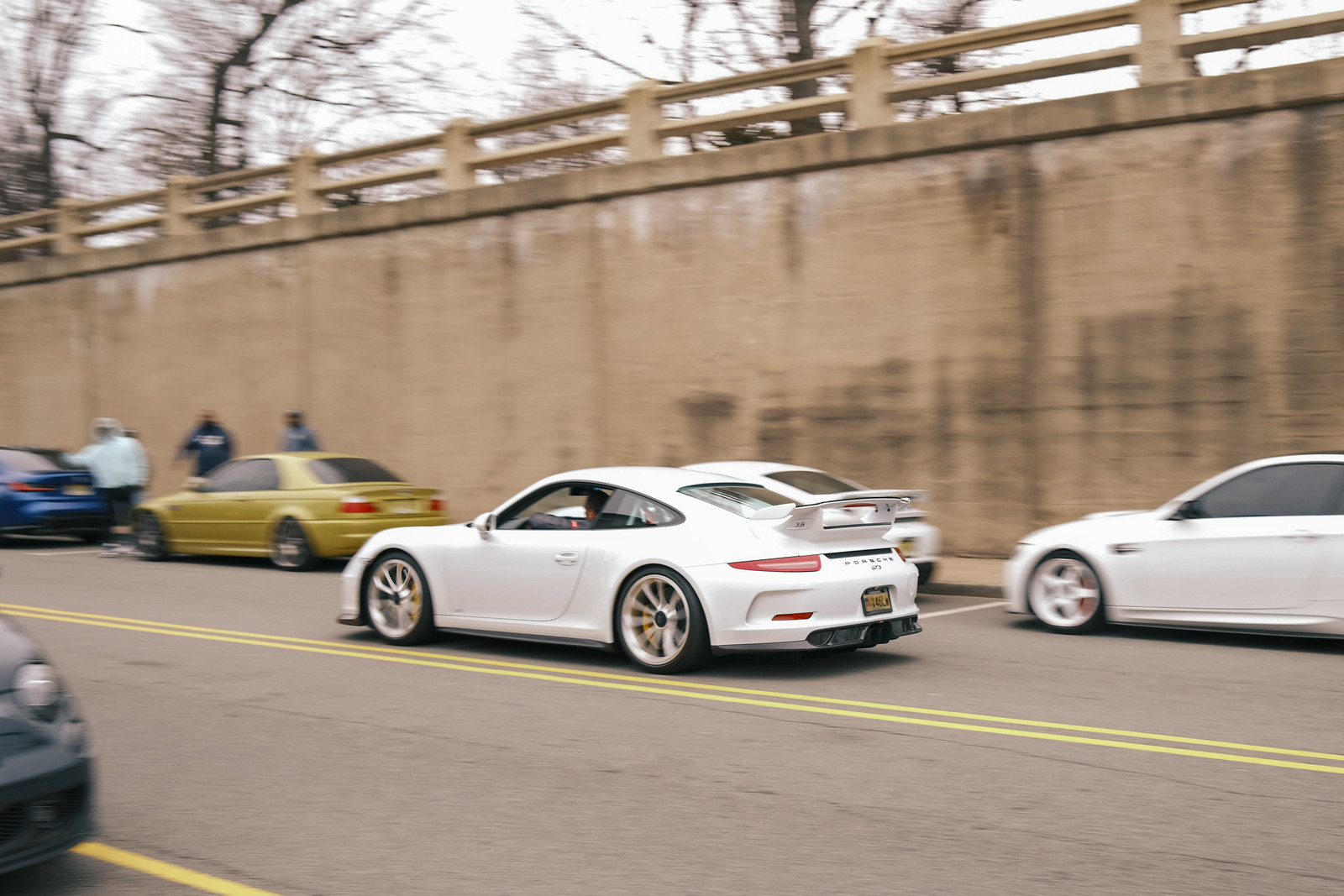The photograph features a dynamic cityscape with six cars on a road, primarily traveling from right to left. Dominating the scene is a white, two-door sports car, likely a Porsche, situated centrally in the frame and facing away from the viewer. This car, equipped with black tires, white rims, a silver brand logo, a yellow license plate, and a distinctive rear spoiler or fin, is positioned on a gray road marked with a yellow double line to its left.

In the mid-ground, there's another white car behind the Porsche, followed by a faint glimpse of a headlight in the bottom left corner. Also, a gold-colored car and another white car are visible, with a blue car further left. A dark blue car is barely visible towards the far left. Three indistinct figures walk along a sidewalk in the background, near the blue and gold cars, dressed in white, black, and blue jackets respectively.

The backdrop features a large, brown wall topped with a brown fence, behind which leafless brown trees extend against a pale white sky. This setting suggests an outdoor scene on a busy city street or causeway, with a cement bridge and railing visible at the top of the image.